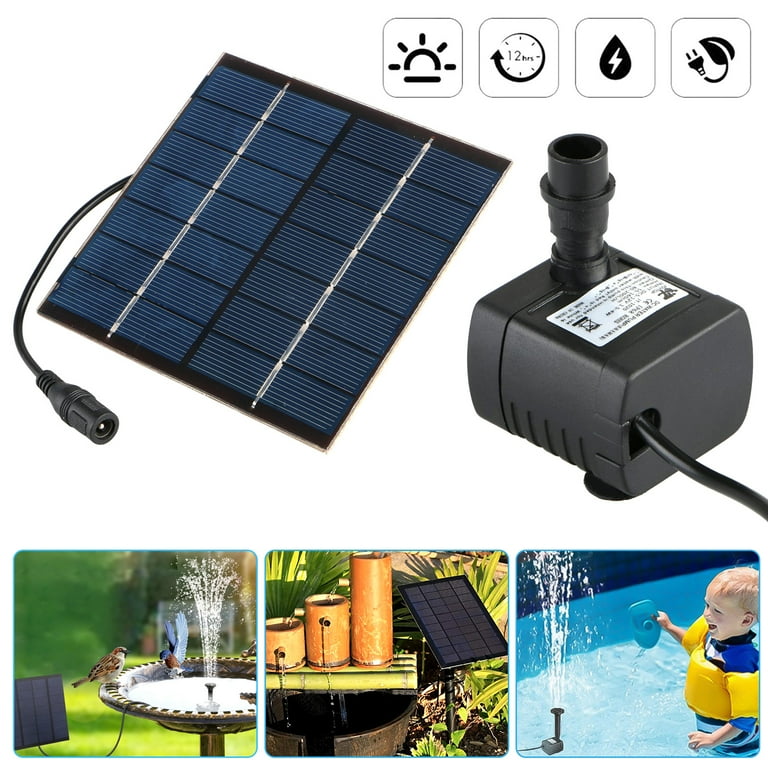The image is a composite of several smaller photos, each showcasing various aspects and uses of a solar-powered fountain. At the top right, four icons in separate boxes highlight different features of the product: from left to right, a sun rising, a clock with "12 hours" indicating operational time, a water drop with an electrical symbol, and a leaf with a power cord, suggesting eco-friendliness. Below these icons, the left side shows a black solar panel with a plug and wire, whereas the right side features a charging outlet, implying that the solar panel powers the fountain.

At the bottom of the image, three separate photos illustrate different applications of the solar fountain. On the left, a solar-powered birdbath shoots water, combining functionality with decorative appeal. In the center, the fountain operates a series of cascading water cylinders, showing versatility in garden decor. The far-right photo depicts a child in a blue shirt with yellow floaters joyfully watching the fountain spray water, showcasing its use as a playful pool toy. This detailed layout emphasizes the fountain's multiple uses—birdbath, garden decoration, and children's pool toy—powered by a sustainable solar panel system.